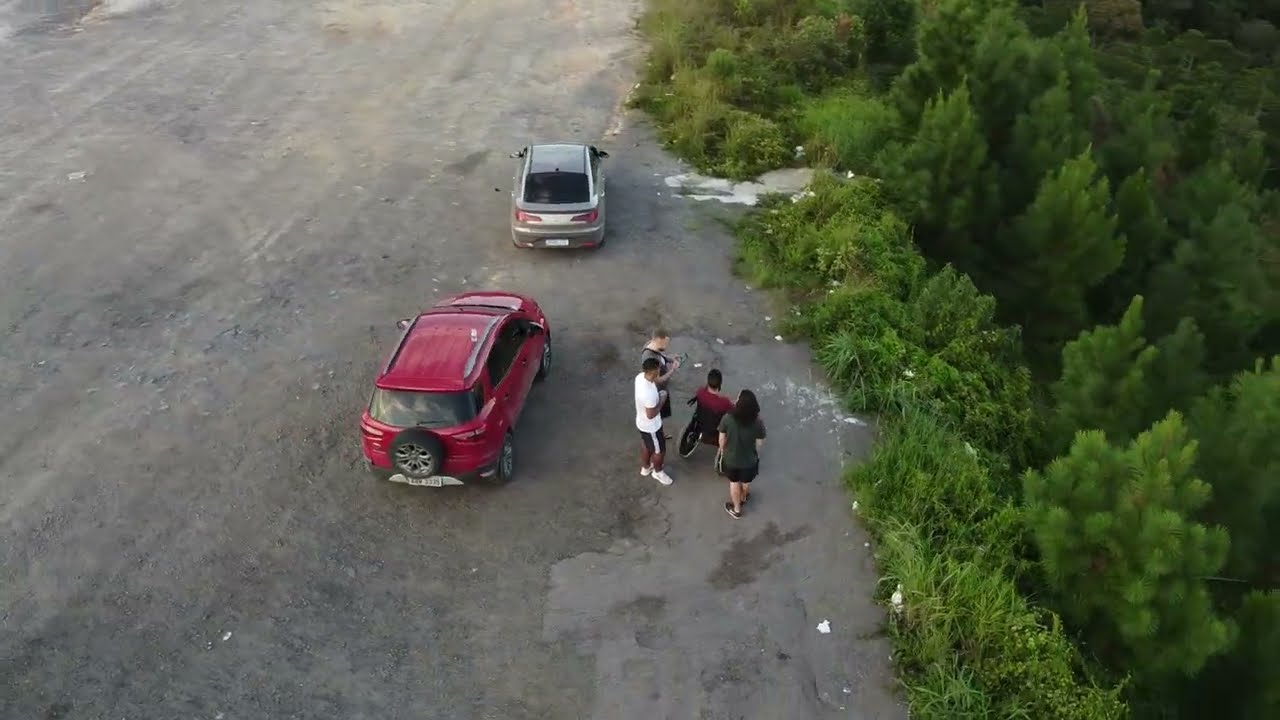This aerial photograph, likely captured by a drone, depicts a dirt and gravel area transitioning into a lush, green ravine. Parked in the dirt are two vehicles: a silver coupe at the top of the image and a red minivan or SUV just behind it, featuring a spare tire mounted on its back. A group of four people are gathered near these vehicles. The group includes a person in a wheelchair wearing a red shirt, situated closest to the vehicles. Adjacent to this individual stands a woman in a black dress and tennis shoes, distinguished by her long brown hair. To her left, an African American male is clad in a white t-shirt, black shorts with white stripes, and white sneakers. Completing the group is a man with brown hair and a gray t-shirt, who appears to be holding a camera with a strap around his neck. The scene is set near the edge of a steep ravine filled with both deciduous and pine trees, accompanied by tall grasses along the border. The left side of the photograph is dominated by a dry, barren landscape with dirt and rocks, while the right side features dense shrubbery and greenery, creating a stark contrast within the image.